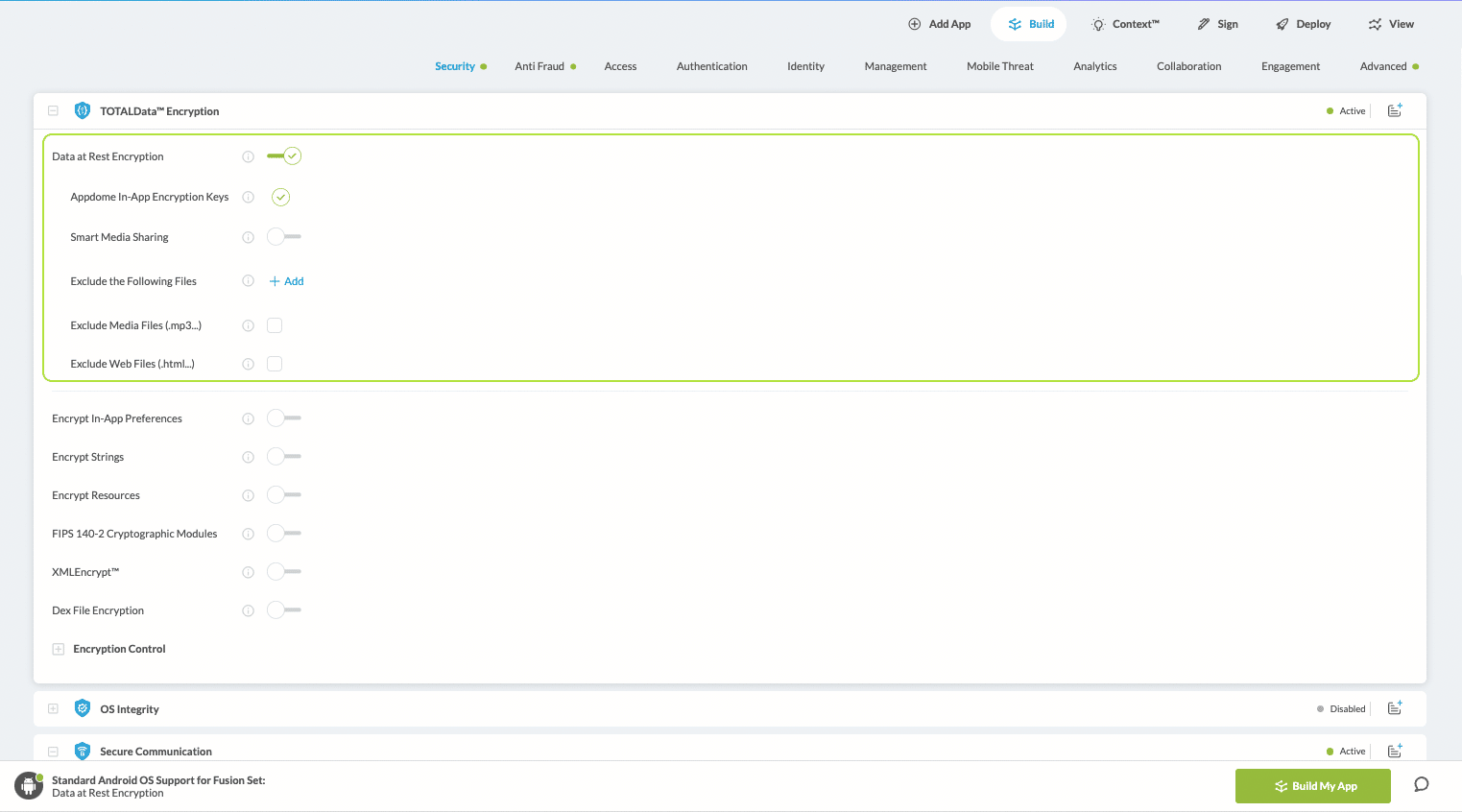The image displays a comprehensive interface layout featuring multiple sections and icons with detailed annotations. 

On the right side, there is a circle with a dark gray plus sign, adjacent to which is the word "App" in dark gray. Beside this, a white oval button displays the word "Build" in blue. Following this are several functionalities listed in gray: "Context," "Sign," "Deploy," and "View." 

The next line highlights "Security" in blue, accompanied by an armored circle symbol. Below this, "Anti-fraud" is mentioned in black (or gray), with a green circle adjacent to it. The term "Authentication" is written in dark gray, alongside terms such as "Identity Management," "Mobile Threat Analytics," "Collaboration," "Engagement," and "Advance," each linked with a green circle.

A white rectangle featuring a dark blue shield with white lines is also visible. Below this, the text "Total Data" is shown in dark gray, followed by "TM" (trademark) and "Encryption." The term "Active" is marked with a green circle.

The section beneath this contains various options such as "App Don't," "App Encryption Keys," "Smart Media Sharing," and several exclusions like "Exclude the following files," "Exclude media files," and "Exclude web files." Additional encryption settings and controls are listed including "Encrypt in-app preferences," "Encrypt strings," "Encrypt resources," "FIPS 140-2 Cryptographic Modules," "AMXL Encrypt," "Dex File Encryption," "Encryption Control," "OS Integrity," "Secure," "Locate," and "Communicate." Each function is meticulously documented to reflect the comprehensive security and encryption measures available in the application.